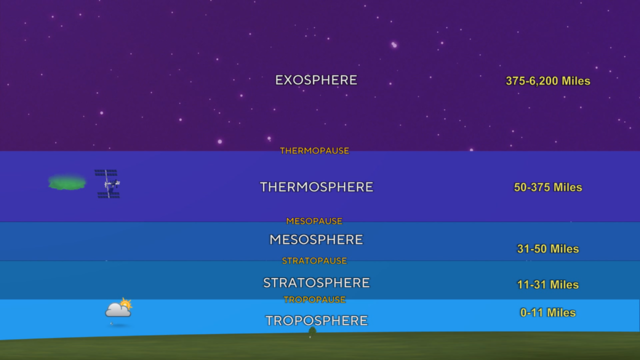The image is a horizontally aligned rectangular graphic depicting the layers of Earth's atmosphere. At the very top, against a dark purple background with white star-like dots, white text reads "EXOSPHERE," with "375 to 6200 miles" in yellow text to the right. Below this, a blue-shaded segment labeled "THERMOSPHERE" in white text occupies the center, featuring a satellite and a pill-shaped device on the left. Above the thermosphere, yellow text spells out "THERMOPAUSE." The thermosphere spans from "50 to 375 miles," indicated in yellow on the right. Further below, another blue section is marked "MESOSPHERE" in white text, with "31 to 50 miles" in yellow to the right. This section transitions into the "STRATOSPHERE," distinguished by a slightly darker blue and labeled with white text, extending "11 to 31 miles" as noted in yellow. The lowest layer is the "TROPOSPHERE," indicated by a light blue color with its range "0 to 11 miles" in yellow text on the right. Between each atmospheric layer, separations are marked by terms in orange text, such as "MESOPAUSE" and "STRATOPAUSE."